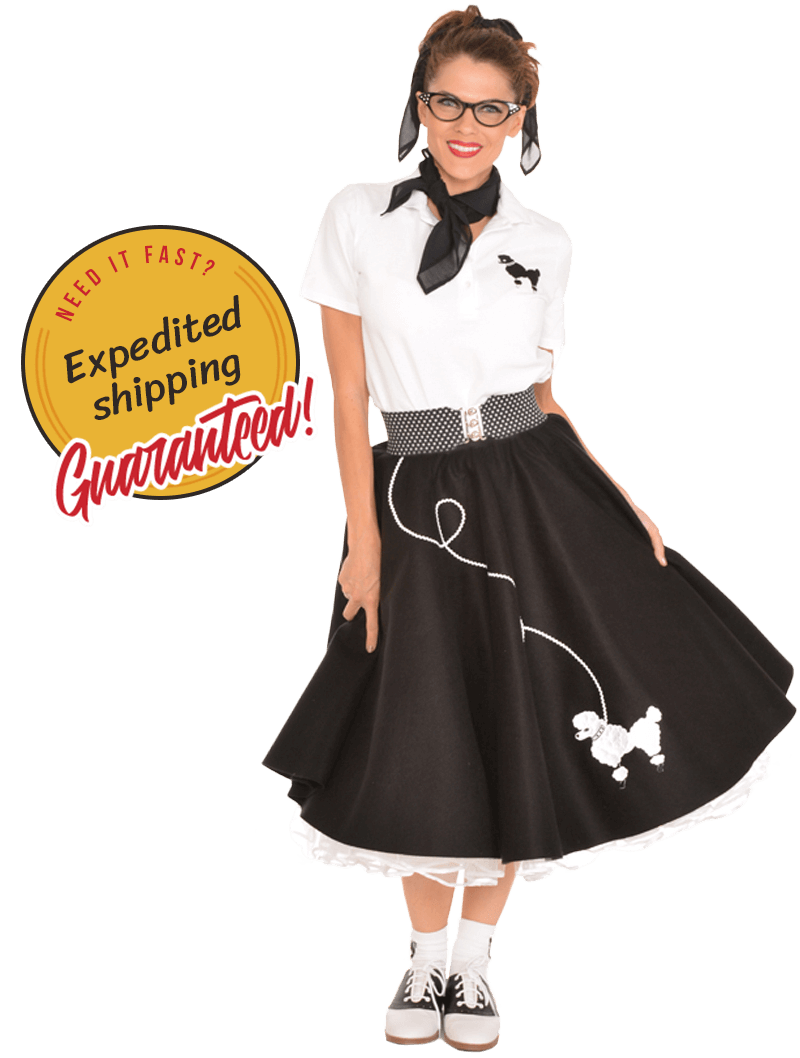In the image, we see a woman dressed in a 1950s-inspired outfit, standing against a stark white background. She wears a white shirt adorned with a black poodle graphic, accessorized with a thin black scarf around her neck and another tied in her hair. Her black poodle skirt, which poofs out with white lace trim sticking out from underneath, features a long leash attached to a white poodle design. She completes her retro look with black and white saddle shoes, white socks, a black and white belt with a silver clip, and black cat-eye glasses. Bright red lipstick accents her smiling face, and she stands with her hands at her sides, holding her skirt. To the left of her, a yellow circle contains the promotional text, "Need it Fast, Expedited Shipping Guaranteed," in red and black letters, with a logo placed above the circle on the top left corner of the image. The overall style and sentiment of the image resemble a vintage advertisement.